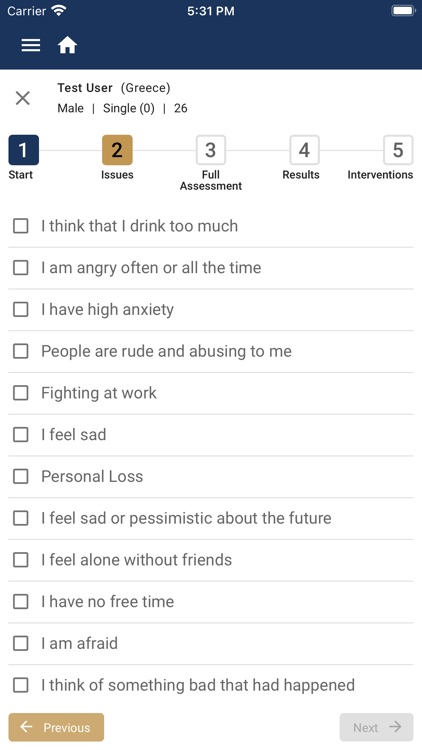This is a mobile screenshot of a test user page for a survey, specifically a user test page. The header at the top of the page is dark blue. On the left side of the header, there is a home icon, and on the far left, a menu icon is located. Below the header, the main page has a white background. At the top, the text "Test User" is displayed in bold, blue print, with "Greece" in parentheses beside it. Directly below, demographic information is provided: "Male, Single" followed by "0" in parentheses and "26," indicating the user's age. On the top left, a large "X" appears next to "Test User," allowing the user to exit the page.

Further down, five numbered tabs stretch horizontally across the page, connected by a thin gray line. These tabs are labeled as follows: "1. Start," "2. Issues," "3. Full Assessment," "4. Results," and "5. Interventions." The first tab, "Start," is highlighted in blue, while the second tab, "Issues," is highlighted in brown. Below the tabs, vertical lines of questions are listed. The first question reads, "I think I drink too much," with checkboxes to the left of each question; none of the checkboxes are selected.

At the bottom of the page, there are navigation bars. On the bottom left, a brown bar is labeled "Previous," and to its right, a gray bar is labeled "Next."